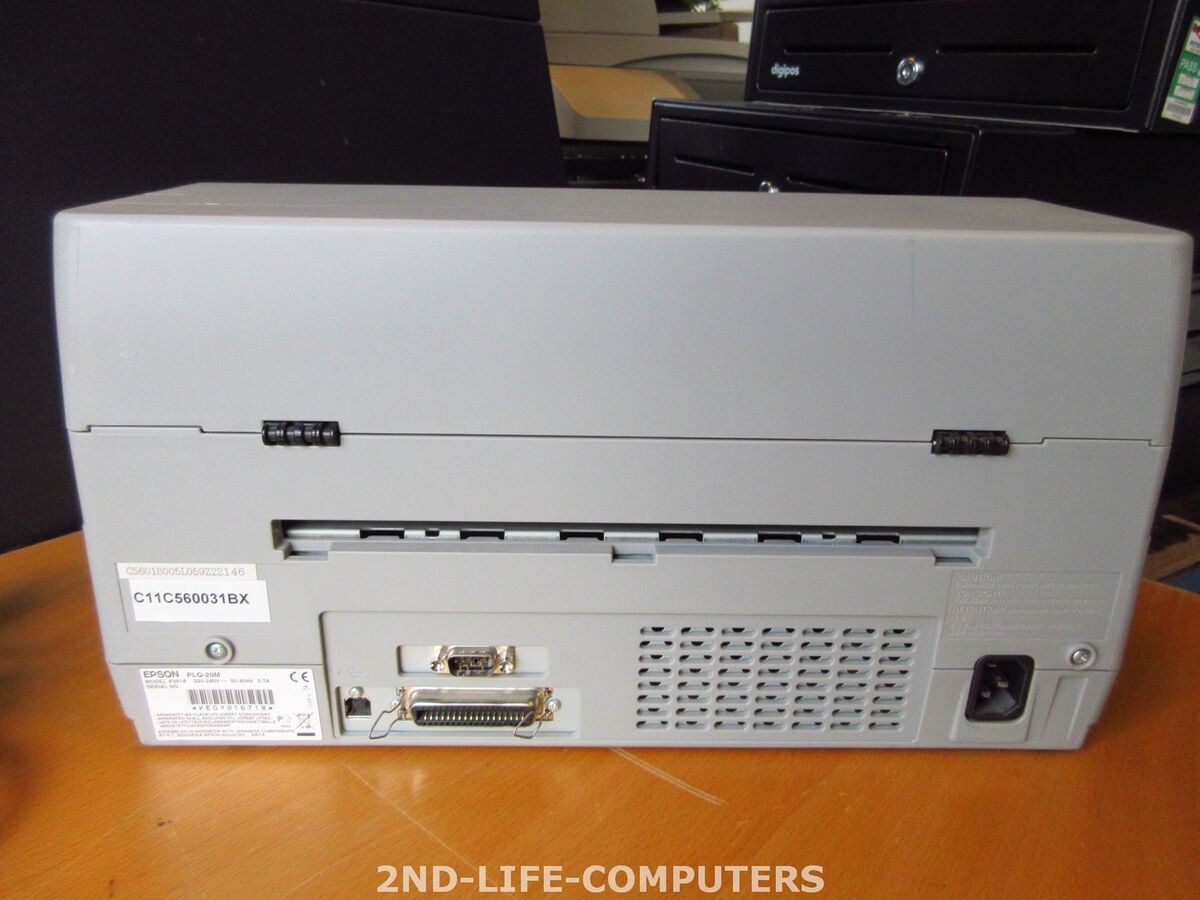The photograph captures the back side of an Epson printer, identified by the label "Epson" in the bottom right and a black serial number C11C560031BX on a white sticker. The printer, which is gray and somewhat resembles a tackle box, sits on a brown wooden table in an office-like setting. The device features various ports, including USB and outlet ports, a ventilation grid, and an indent slit at the bottom. In the background, there is a computer monitor and possibly another printer or copy machine, though the scene is quite dark. The image also includes a watermark at the bottom center that reads "Second Life Computers," suggesting recycled or refurbished equipment.